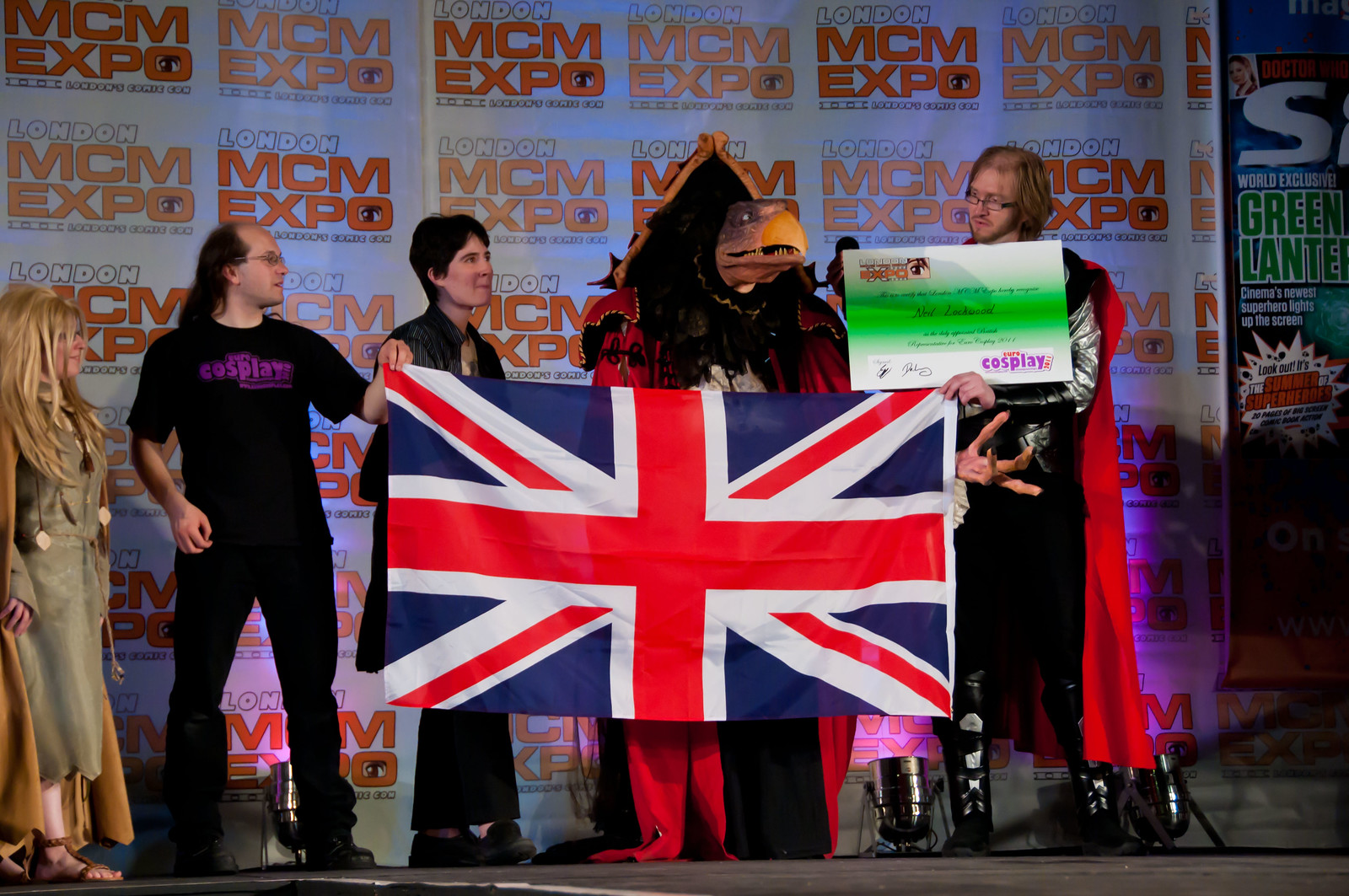This detailed color photograph captures a lively scene at a London MCM Expo event. The backdrop is adorned with a repeating logo that reads "MCM Expo" in bold red letters beneath a larger "MCM," arranged in a grid pattern both horizontally and vertically. 

Centerstage, five individuals stand side by side, partially concealed by a large British flag they hold collectively. Each person is distinct in their attire, most of which are themed in elaborate costumes suggestive of a cosplay competition or presentation.

Starting from the left, a woman with shoulder-length blonde hair wears a robe and sandals. Beside her is a man dressed in a black t-shirt with purple lettering that spells "cosplay" and black pants; he also has dark-framed glasses and his hair cascades behind his ears. He shares the responsibility of holding the flag with the person next to him, a woman with dark hair, dressed entirely in black. 

At the center is a striking creature-like figure with a large yellow beak and an elaborate triangular black headdress. This individual dons a combination of white and black robes, adding to the impressive nature of their costume.

To the right of this figure stands a man with long fair hair, wearing dark-framed glasses and a red cape. He holds up a sign that features sections of green and purple, prominently displaying the word "cosplay" in purple text. 

All the individuals are positioned in front of a vivid backdrop, collectively contributing to an engaging and dramatic tableau, likely signifying their participation in a cosplay contest or presentation.